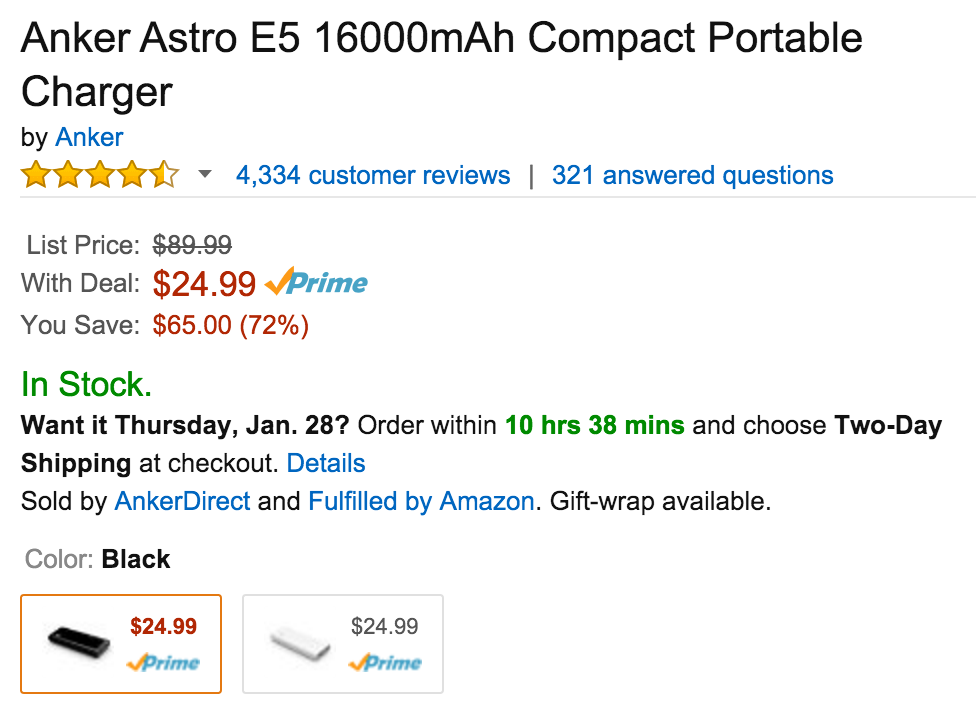**Detailed Product Information for Anker Astro E5-16000MAH Compact Portable Charger**

The screenshot captures a detailed Amazon product page for the "Anker Astro E5-16000MAH Compact Portable Charger." The page is set against a white background, with the product title displayed prominently at the top in black font, accompanied by the brand name "Anker" in blue font.

Below the product title, customer ratings are shown: a row of yellow stars indicates a 4.5 out of 5-star rating, based on 4,334 customer reviews, which is clickable and presented in blue font. There are also 321 answered questions available, also in blue font and clickable.

A gray line separates the above information from the pricing section. The original list price of $89.99 has a slash through it, indicating a sale. The discounted price of $24.99 is highlighted in bold red font, accompanied by the gold Prime checkmark and the word "Prime" in blue font. Directly below, the caption notes that buyers save $65, which translates to a 72% discount.

Availability is promptly stated as "In Stock" in bold green font. Shipping details follow: to receive the item by Thursday, January 28th, one must order within 10 hours and 38 minutes, with the countdown displayed in green font, and select two-day shipping at checkout. Further shipping details can be accessed via a clickable blue link labeled "Details."

Additionally, the product is sold by "Anker Direct" and fulfilled by Amazon, both indicated in blue font, along with an option for gift wrapping. The charger is available in two colors: black and white. Both versions are priced at $24.99 and include the Prime logo underneath. The black version is currently selected, evidenced by a mustard-colored box around its image and pricing information.

This comprehensive snapshot provides potential buyers with clear and detailed information about the Anker Astro E5-16000MAH Compact Portable Charger, helping them make an informed purchase decision.